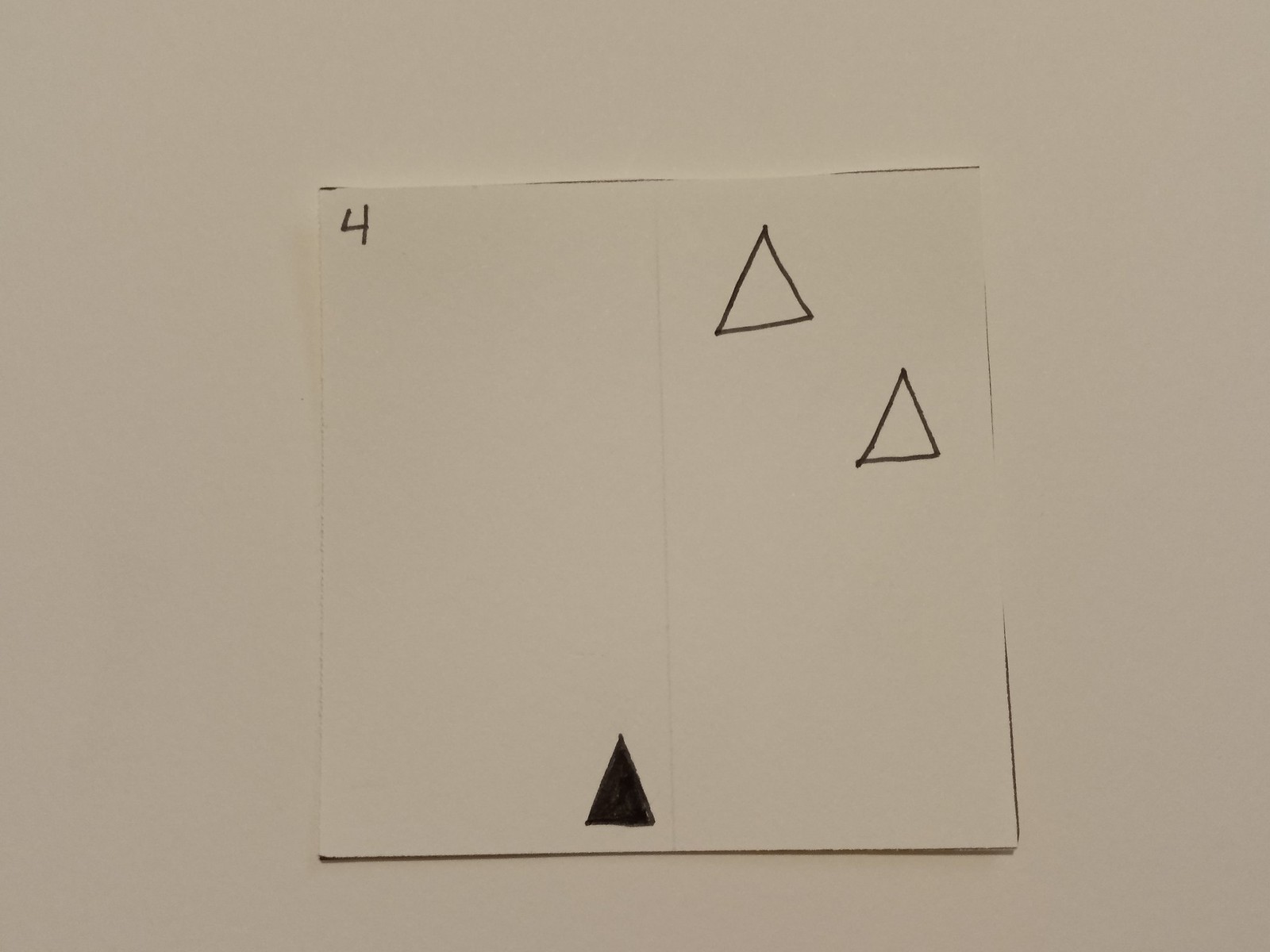This image features a predominantly white composition. The background resembles white paper, establishing a minimalistic and clean aesthetic. Central to the image is a perfectly square piece of white paper, distinguishable by a subtle shadow that indicates it is a separate layer positioned atop the background.

In the upper right corner of this square paper, the number "4" is inscribed in black ink. A prominent vertical fold or crease runs down the exact middle of the square, extending from the top edge to the bottom edge, clearly dividing the square into two equal halves.

Positioned in the bottom right corner, on the left side of the fold, is a solid black triangle. Adjacent to the fold on the right side, the geometric theme continues with a simple outlined white triangle in the upper left corner. Directly below this, slightly offset to the right, lies another triangle consisting only of a black outline. The interplay between these elements adds a subtle complexity to the otherwise monochromatic and minimalist design.